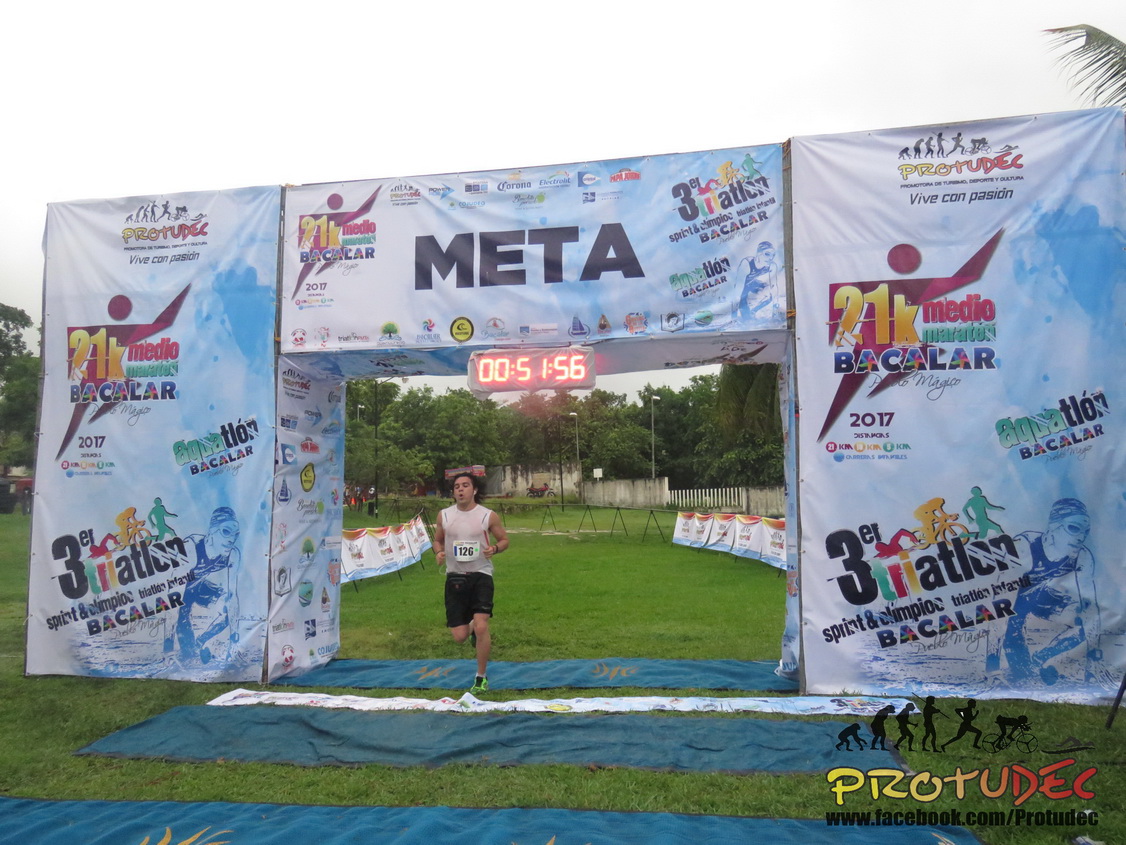In this image, a man is captured mid-run at the finish line of a race, positioned centrally within the frame. He is wearing a tan sleeveless t-shirt, black shorts, and neon yellow tennis shoes. A bib with the number "1126" is pinned to his shirt. He is approaching an archway structured from three rectangular sections—a large central one flanked by two smaller supports. At the top of the archway, there are various logos and inscriptions including "3ER Triathlon," "Sprint," "Olympic Triathlon Baccalaureate," "META," and "Pro2Dick," with the last also appearing at the bottom right corner along with a web address, www.facebook.com/Pro2Dick. A red LED timer is displayed on the lower section of the central rectangle, reading "00:51:56." Surrounding the finish line are several blue tarps laid out on a grassy surface. The setting is outdoors, and the scene is bathed in a vibrant array of colors, including green, blue, yellow, red, orange, black, white, tan, purple, gold, and pink. Several spectators can be glimpsed in the background, observing the event.